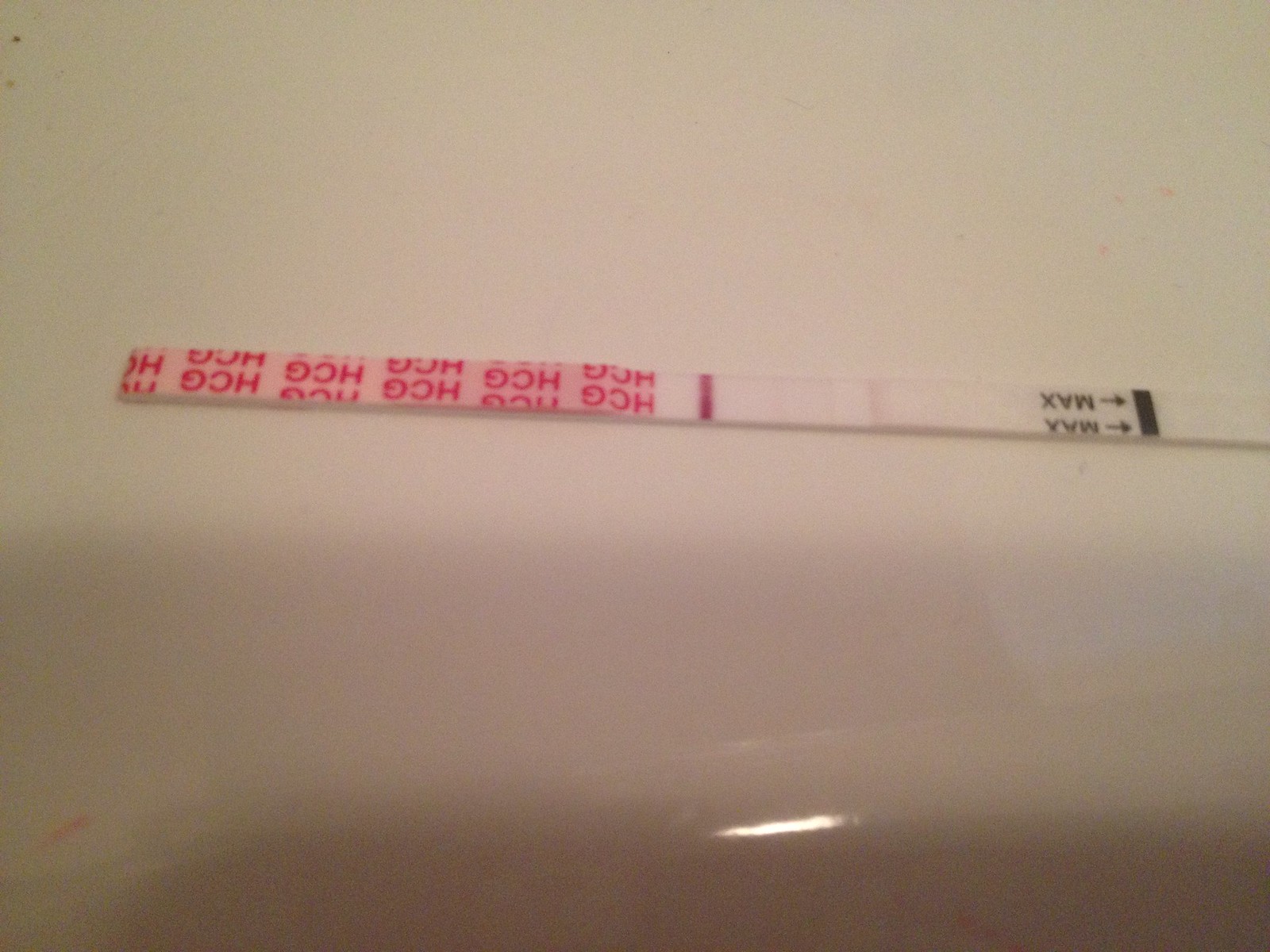The image, a horizontally oriented photograph resembling a home snapshot, features a close-up of a white countertop. Centered prominently on this surface is a pregnancy test strip. The test displays the label "HCG" on the left side, along with one thick line and a faint second line, indicating a positive result. The remainder of the strip is predominantly white. On the right side of the test, the word "MAX" appears twice, accompanied by two lines pointing right towards a small bar.